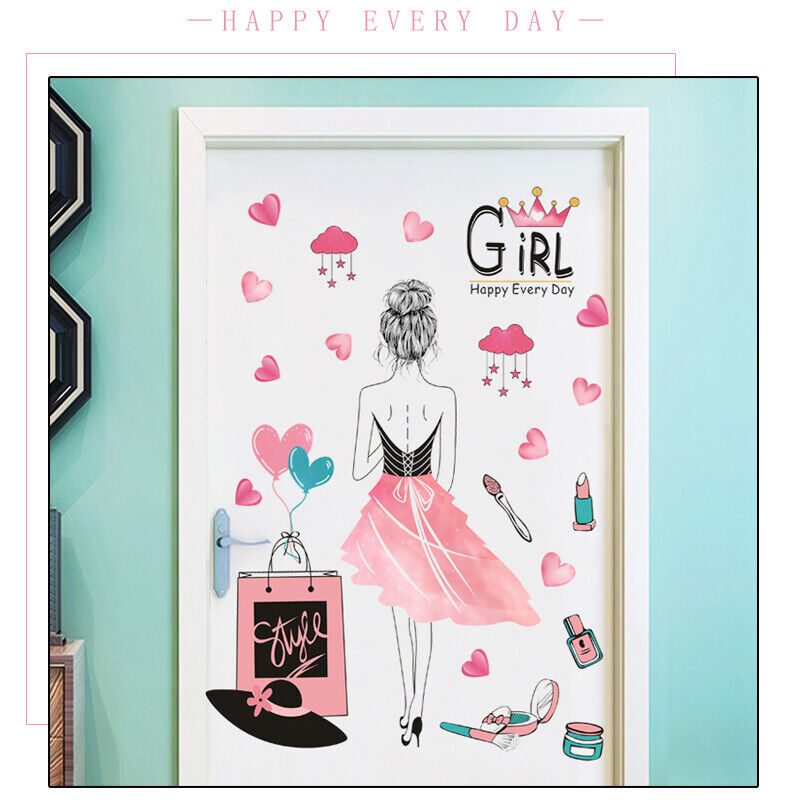The image depicts a highly detailed decorative door print designed to resemble a framed piece of wall art. The door is adorned with a white background and features a prominent illustration at its center: the back of a woman wearing a low-cut, backless dress. The dress has a flowing pink skirt and a black top, and the woman is accessorized with black stiletto heels and her hair pulled up into a bun. 

In the upper right corner of the print, the text reads "Girl, Happy Every Day," accompanied by a pink crown with yellow accents and pink clouds from which stars dangle. The print is further embellished with numerous pink hearts, as well as some in aqua blue. Along the bottom left side, there is a pink shopping bag marked with the word "STYLE" in cursive, paired with a black wide-brimmed sun hat decorated with a pink ribbon and flower. Additionally, scattered cosmetic items in pink and blue hues are interspersed throughout the design, complementing the overall girly and fashionable theme.